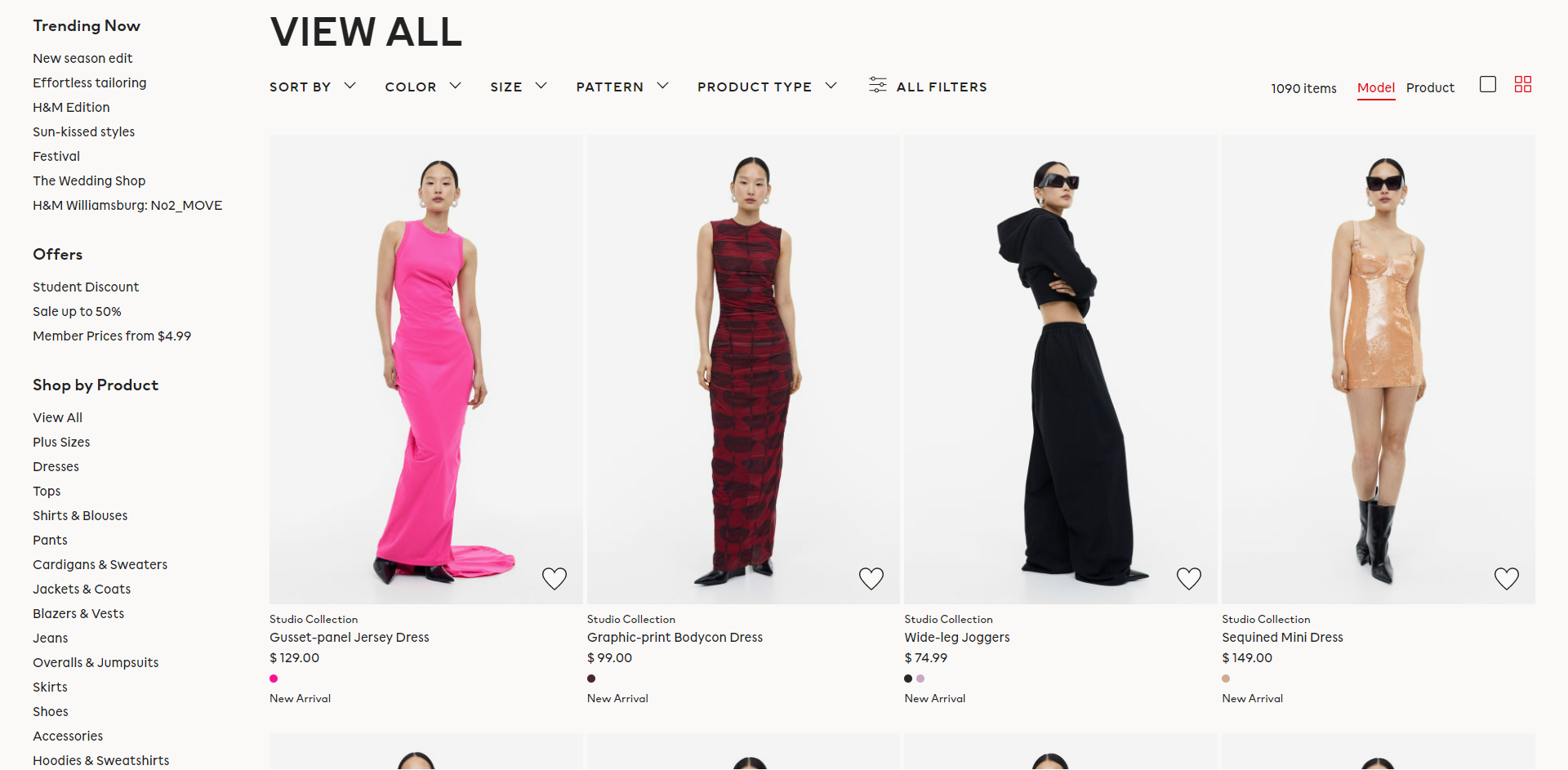The rectangular image depicts a screenshot of an online shopping website where someone is searching for a dress. The layout includes a thin column on the left side of the webpage featuring menu options and categories, while the larger, main body of the website is situated to the right. 

The left column starts with the heading "Trending Now," followed by several subcategories: "New Season Edit," "Effortless Tailoring," "H&M Edition," "Sun-Kissed Styles," "Festival," "The Wedding Shop," "H&M," and "Williamsburg." Below these sections are additional categories labeled "Offers" and "Shop by Product." The background color of the entire page is an off-white shade.

In the main body of the website, the topmost section prominently displays the title "View All." Directly beneath this title is a navigational menu including options such as "Sort by Color," "Size," "Pattern," "Product Type," and "All Filters," which extends about halfway down the page. 

To the far right of the screen, the page indicates there are "1090 Items" available, followed by labels "Model" and "Product." Below this, the website showcases four images of different clothing items: a pink dress, a red and black dress, a black outfit consisting of pants and a halter hoodie, and a short beige dress.